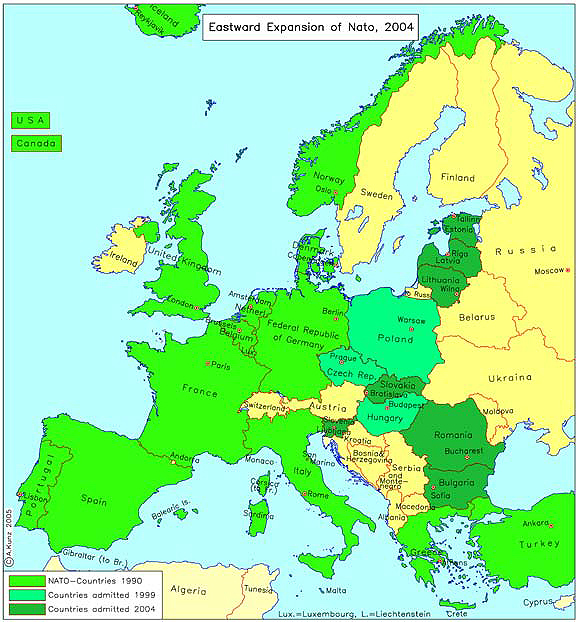The image showcases a detailed map of Europe titled "Eastward Expansion of NATO 2004," prominently displayed at the top in black text within a white rectangle. The map features countries marked in different colors, indicating their NATO membership status. The countries that were part of NATO by 1999, including Greenland, Iceland, the United Kingdom, Norway, the USA, Canada, Germany, France, Italy, Spain, Portugal, and Turkey, are shaded in bright green. Countries admitted to NATO in 1999, such as Poland, the Czech Republic, and Hungary, are displayed in a bluish-green color. Additionally, countries that joined NATO in 2004, including Lithuania, Bulgaria, Romania, Slovakia, Latvia, and Estonia, are highlighted in a dark green shade. 

The map also has small black font labels for the country names and small orange stars indicating the capitals. The surrounding waters are depicted in a light blue hue. A legend is situated in the bottom left corner, providing a clear key for understanding the color distinctions: NATO countries in bright green for 1999, bluish-green for those admitted in 1999, and dark green for those admitted in 2004. Other notable countries like Russia, Ukraine, and Belarus are labeled on the map as well, enhancing the comprehensive depiction of NATO's eastward expansion.